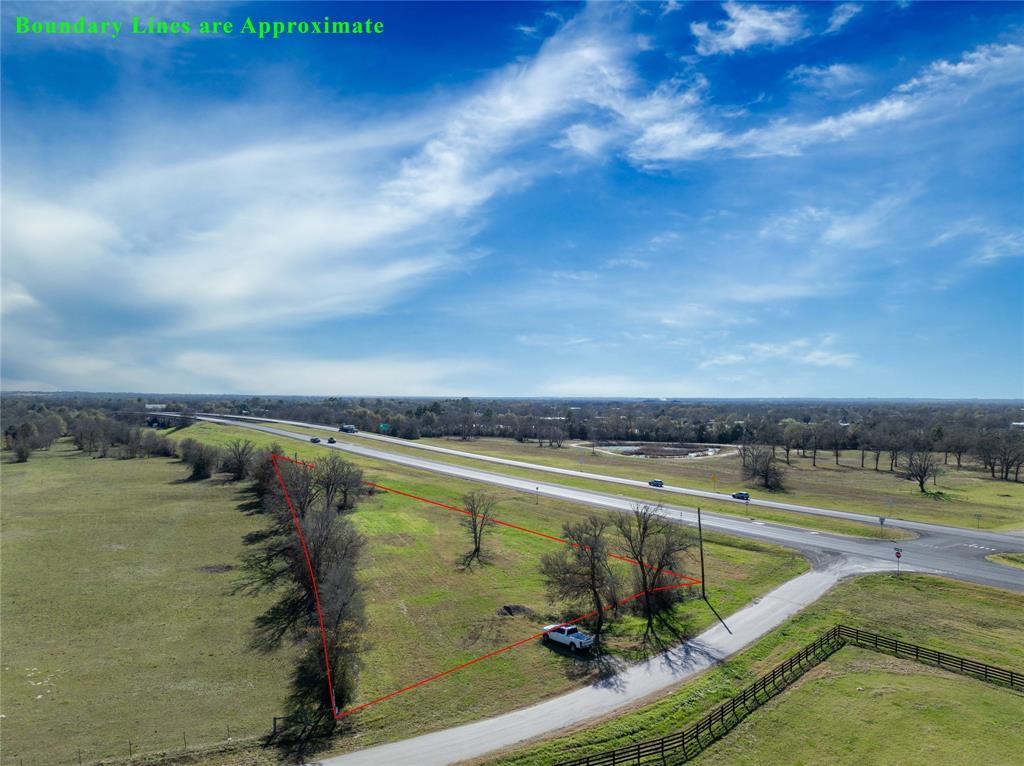This outdoor photograph captures a detailed aerial view of a residential town. In the upper left corner, a vibrant green font reads "Boundary lines are approximate." Below this text, the sky appears a bright blue adorned with delicate, wispy white clouds. Moving downward, the image showcases the residential area, characterized by intersecting four-way streets and several cars traversing these roads.

Near the bottom left of the image, slightly off-center, a grassy area marked by a red triangle stands out. This area contains a few scattered trees and is bordered by a white pickup truck parked near the outlined boundary. Across the street from this marked triangular area, a fenced-in zone is visible, enclosed by what appears to be either a black or wooden fence.